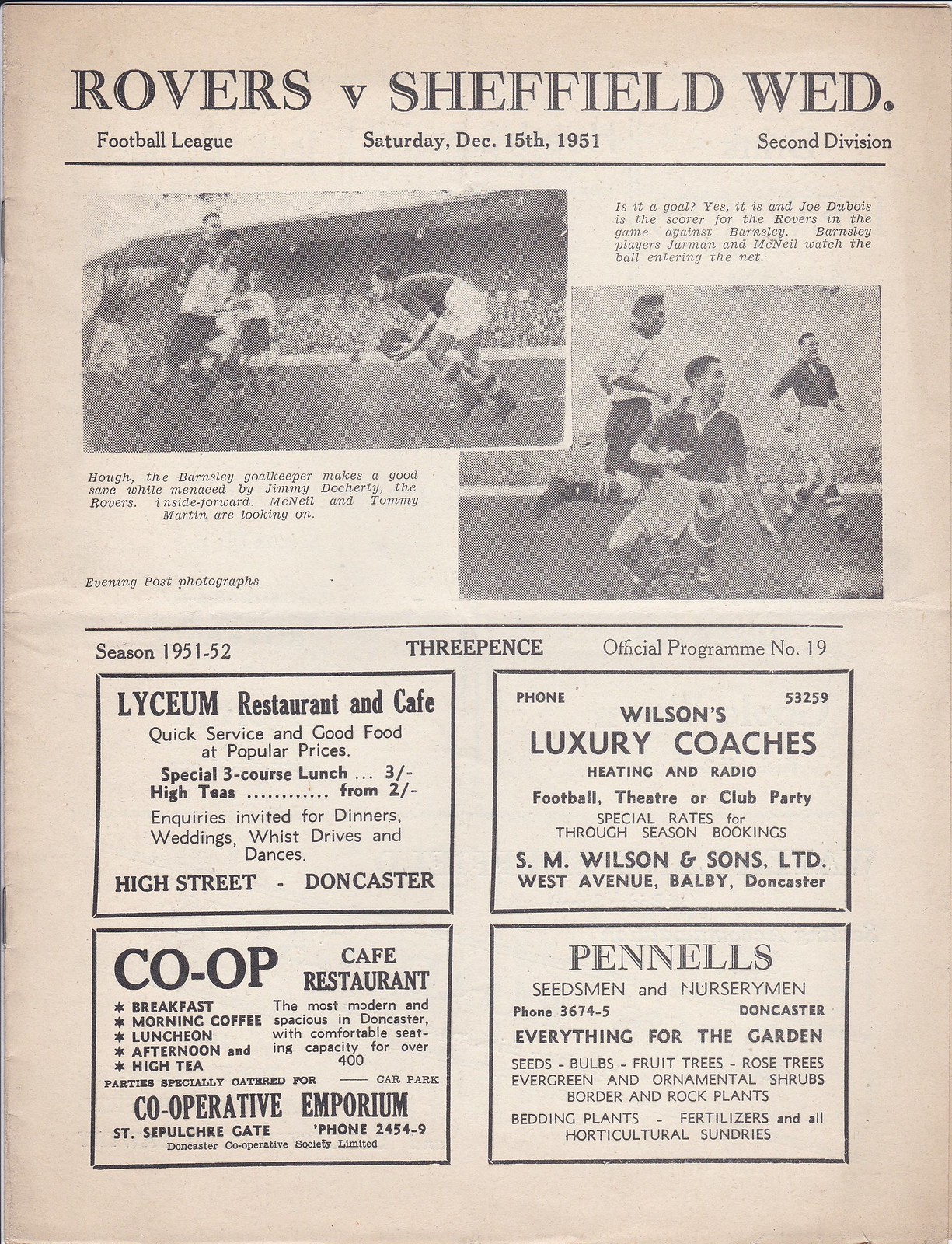The image depicts a single page from an old football-related publication, possibly a newspaper or football program, dated Saturday, December 15th, 1951. The main header reads "Rovers vs. Sheffield Wednesday" with additional text confirming it is a Football League match in the 2nd Division. The page features black-and-white photographs of football players in action and has visible staple marks on the far left side. The background of the page appears to have aged, showing a pinkish tint. Below the photos are four square advertisements promoting local businesses, including Wilson's Luxury Coaches offering heating and radio-equipped coaches for various events, the Lyceum Restaurant and Cafe with quick service and good food at popular prices, the Co-op Cafe and Restaurant, and Pinnell's Seedsmen and Nurserymen, which offers a variety of garden supplies. The ads and the content suggest this is a historic document from the early 1950s showcasing a significant local football match.